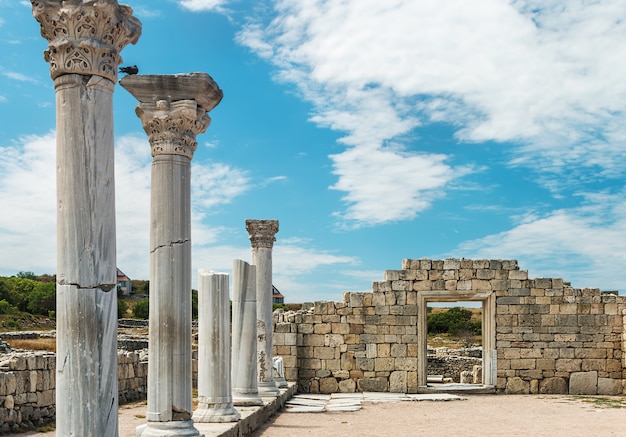The image depicts the ruins of an ancient Greek city, bathed in daylight under a blue sky scattered with white clouds. Dominating the left side of the image are five Greek-style columns: two almost entirely intact while the remaining three are broken off roughly at their midsections, and all show signs of wear and cracks. These columns stand in front of a partially reconstructed stone wall made up of rectangular blocks, with only about four columns of the original wall remaining. Further to the right, a fragmented building wall stands, identifiable by its open doorway devoid of a door. In the backdrop, partially obscured by the columns, are verdant green hills with patches of brown soil visible. The ground in front of the columns and buildings is a light brown, interspersed with sparse patches of green grass. Notably, a bird perches atop one of the columns, adding a touch of life to the serene and historical scene.